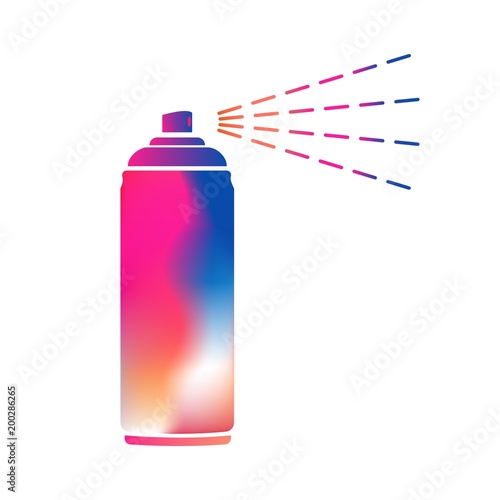The image is a detailed digital illustration of a colorful aerosol spray can set against a solid white background, with "Adobe Stock" and the number "200286265" printed vertically in the lower left corner. The can is upright and facing right. It features a diverse blend of colors: the left part of the can transitions from dark pink to light orange towards the bottom, the right part shifts from dark blue to white and ends in a dark tan at the bottom right. A wavy line vertically divides these hues, creating a tie-dye effect where the colors blend and melt into each other.

The top of the can, including the spray button, is shaded in dark bluish-purple, with the nozzle appearing dark pink. Emanating from the nozzle are four series of dashed lines, representing the spray. These lines are horizontally oriented but vary slightly in angle, with two sets angled upward and two sets downward. The dashes start as orange and transition through pink, purple, and blue, matching the can’s colorful palette. This vibrant spectrum emphasizes the animated spray effect from the nozzle, giving a dynamic and artistic presentation to the illustration.